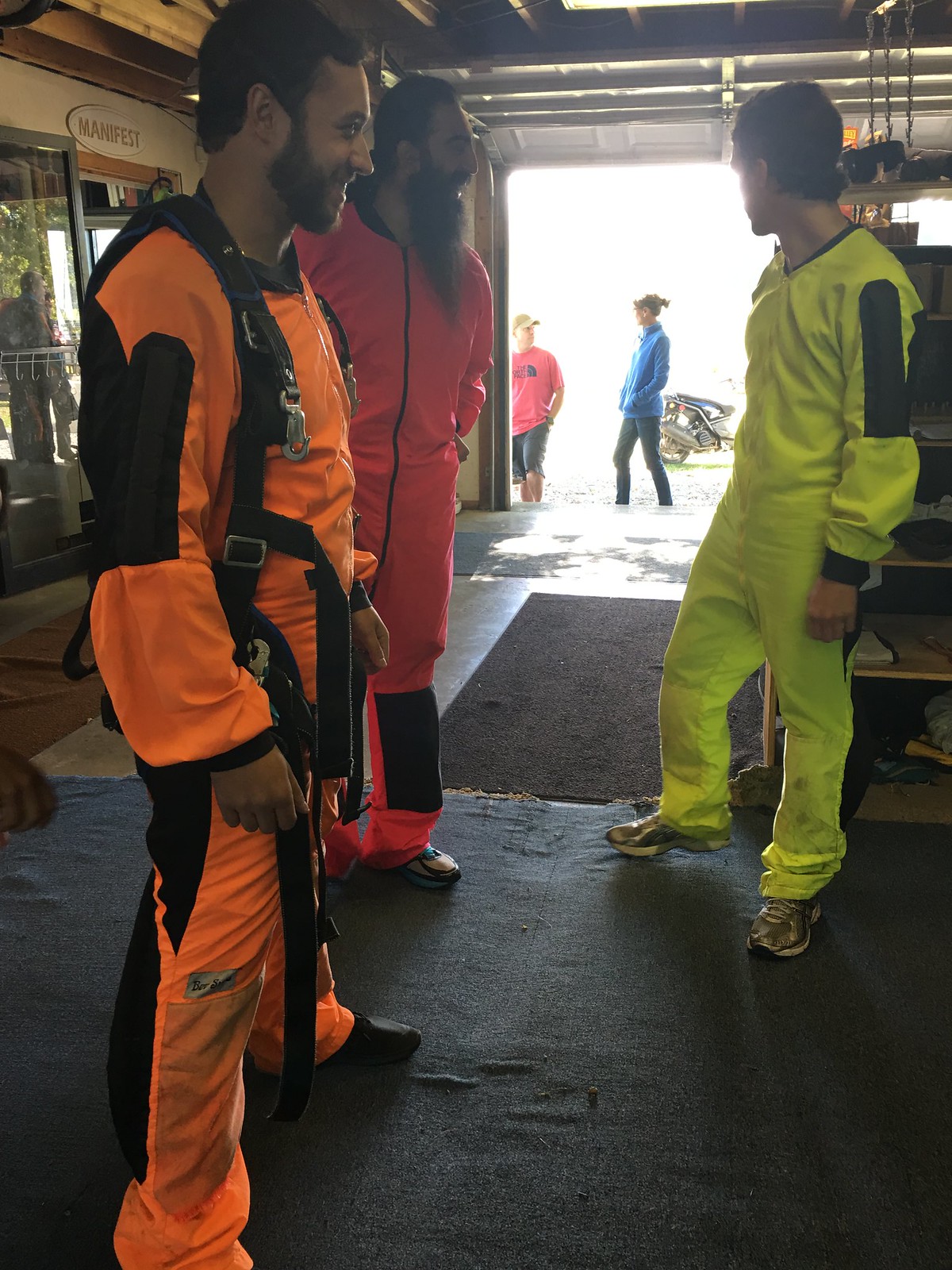This photo shows three men in colorful jumpsuits, possibly preparing for a skydive, inside a spacious garage with a sign reading "Manifest" over the door, suggesting a check-in or office area. The man on the left is dressed in a bright orange jumpsuit with black accents and a black harness, paired with black sneakers and a black backpack with blue details. He has a short beard. Next to him, slightly towards the center, is a man with a long beard, wearing a red jumpsuit with black patches on the shins. On the far right stands a clean-shaven man in a neon yellow jumpsuit with a black band on his left arm, also wearing sneakers. The background reveals an open garage door with bright sunlight streaming in, partially illuminating a motorcycle outside. Two additional people are visible: one in a blue shirt and blue jeans, and another in a red t-shirt and blue jean shorts, both engaged in conversation. A blue carpet lies beneath the men, transitioning to a brown carpet behind them.